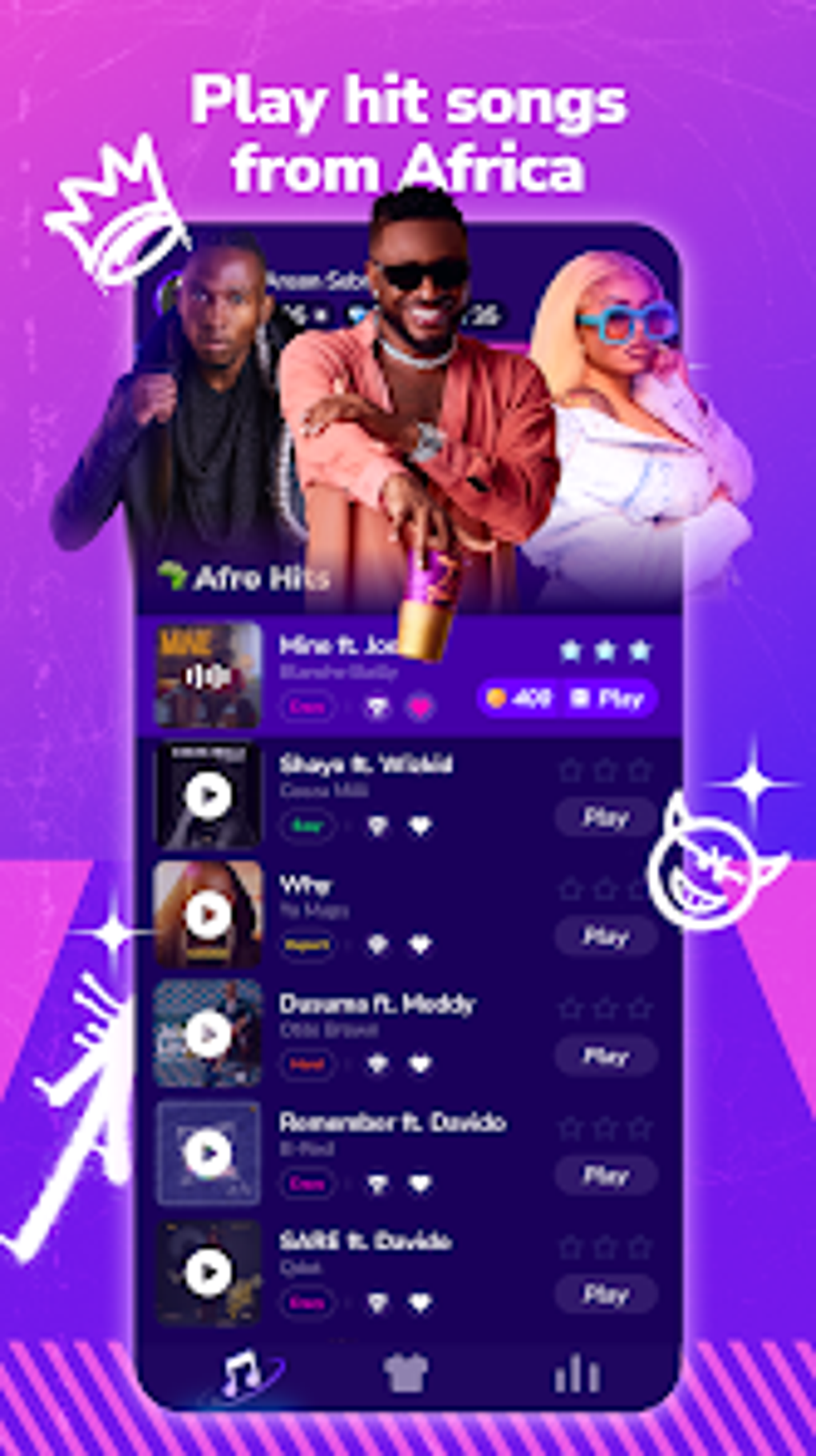A vibrant rectangular image features three African-American individuals set against a purple hued backdrop. Shades of purple, including a purplish-blue and medium purple, blend into the background. At the top, the text "Play Hit Songs from Africa" is prominently displayed in white. In the foreground, two men and one woman stand together, with the man in the center positioned slightly forward, sporting stylish black sunglasses. To his right, a woman with sleek, straight blonde hair parted in the middle, wears blue-rimmed glasses. At the bottom, a slightly blurred section lists the names of artists or songs, accompanied by small images to their left, with the word "Play" appearing to the right of each entry.